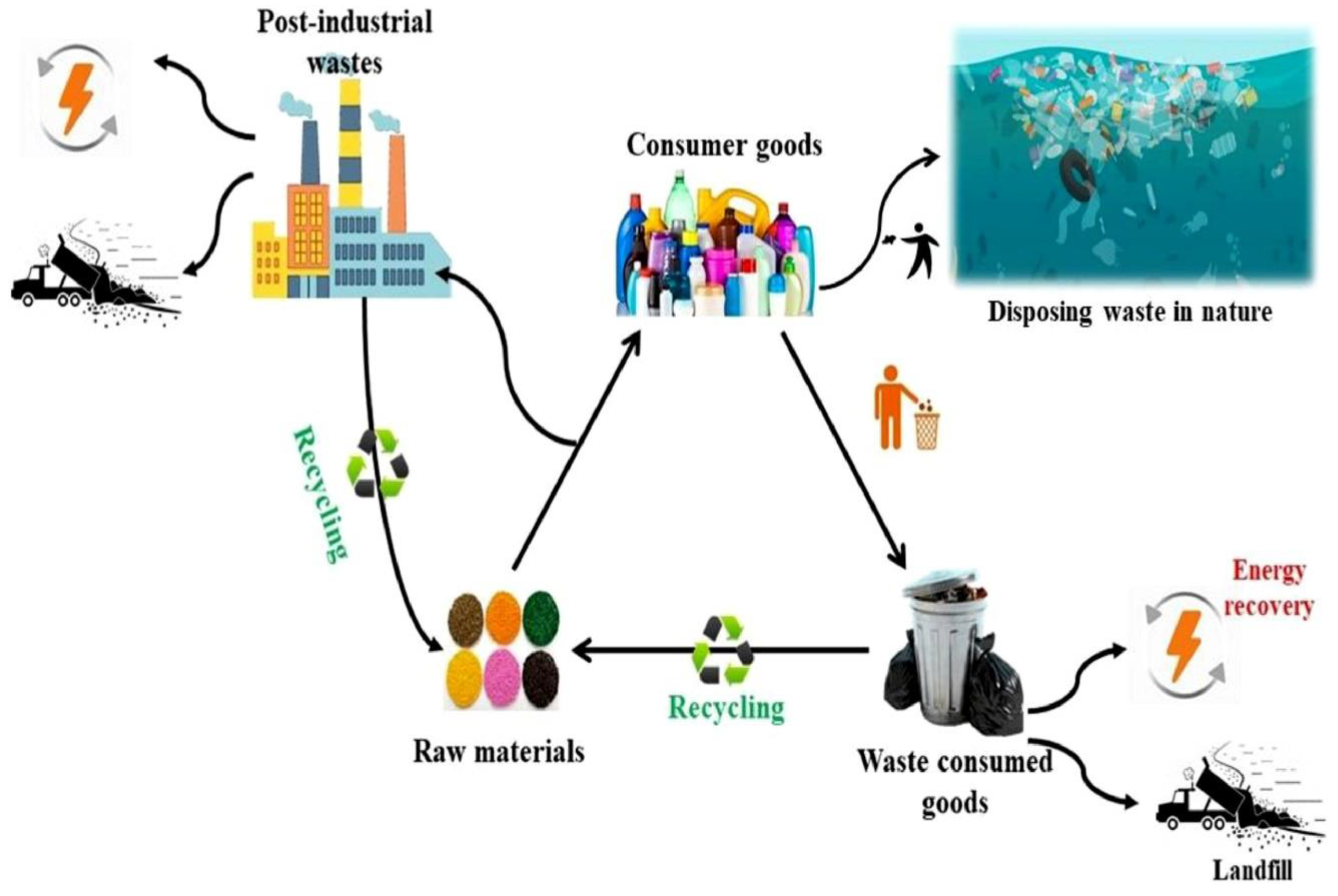This vibrant and intricate mixed-media flowchart illustrates the lifecycle of consumer goods, emphasizing the cyclical nature of production, consumption, disposal, and recycling. At the heart of the diagram are consumer goods, represented by images of bottles and laundry detergents, which highlight everyday items derived from raw materials. The chart traces these materials' journey from post-industrial waste factories, depicted with smokestacks and pollution, to consumer use where goods can either be disposed of in nature, shown by waste in the ocean, or placed in waste bins that lead to landfills or energy recovery.

Arrows connect these stages, demonstrating the continuous flow of materials: raw materials mined by trucks (shown on the left-hand side) feed into factories to create plastic goods and energy (including gasoline), which are then used by consumers. Post-use, the goods either pollute the environment or get processed in landfills or recycling plants, which feed back into the industrial production cycle. The diagram's high use of colors—pinks, blues, yellows, browns, and oranges—makes it eye-catching, but also busy and somewhat confusing, with numerous arrows indicating the complex back-and-forth processes. The white background starkly contrasts with the colorful and diverse graphical elements, combining real pictures with clip art to effectively communicate the messy reality of the consumer goods lifecycle.